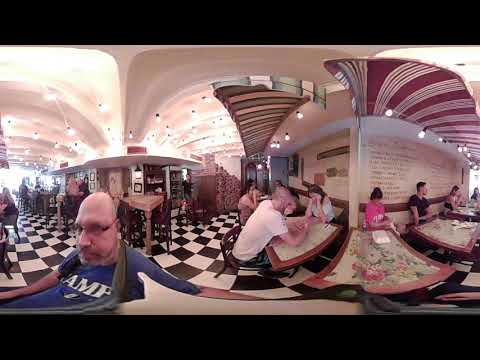The image depicts the vibrant interior of a bustling restaurant, characterized by its bright lighting and numerous decorative details. The photograph has been edited with a slight skew, adding a unique perspective to the scene. The restaurant's floor features a black and white checkerboard pattern, while the ceiling above showcases strings of light bulbs hanging over red and white striped awnings. 

Central to the image are several tables with patrons seated, some of which are adorned with pink flowers and yellow daisies. A man appears in the foreground, taking a selfie. He is a Caucasian man in his 40s with a bald head, glasses with plastic frames, a beard, and wearing a blue T-shirt that reads "AMF" alongside a green scarf.

Towards the back, there is a distinctive bar area resembling a trolley car, attended by a single person. The lighting within the restaurant is enhanced by numerous bulbs, contributing to a lively atmosphere. The color palette includes black, yellow, tan, red, blue, white, and green, all blending to create a warm, inviting environment indicative of a mid-day setting.